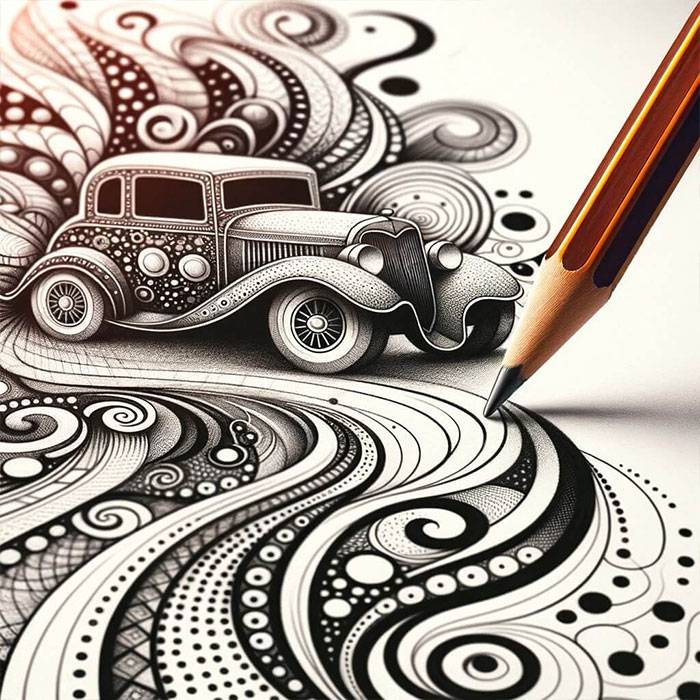This black and white image captures an intricate pencil drawing in progress, as indicated by a large, fully sharpened brown pencil touching the paper from the top right corner. The focal point of this artwork is a vintage car reminiscent of a 1920s or 1930s Model T, though the artist has softened its features, giving it sleeker, rounder edges and fenders. The car, facing right, displays embellished designs, including shaded windows. Surrounding the car and extending throughout the image are psychedelic patterns comprised of swirls, circles, dots, diamonds, and cones. These designs, some filled in, create a dynamic effect that makes parts of the drawing appear three-dimensional, especially as they shoot from the back of the car and swirl around the composition, contributing to the detailed, almost life-like representation.